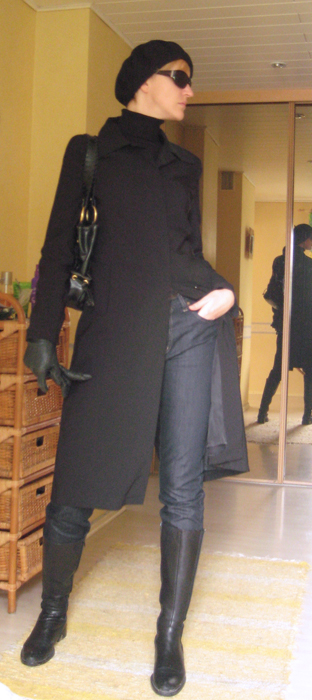In this stylish indoor photograph, a Caucasian woman named Maykenik, known for her fashionable poses on Flickr, stands confidently on a rug, possibly in a bedroom. She wears a long black coat that reaches her knees, paired with dark blue or black jeans and knee-high riding boots. Her outfit is accentuated with black leather gloves—one worn and the other held—along with a black and gold shoulder bag. A black beret and dark sunglasses complement her short blonde hair, completing her chic look. She stands next to a wicker multi-drawer cabinet, with sliding glass mirror doors reflecting the scene in the background.